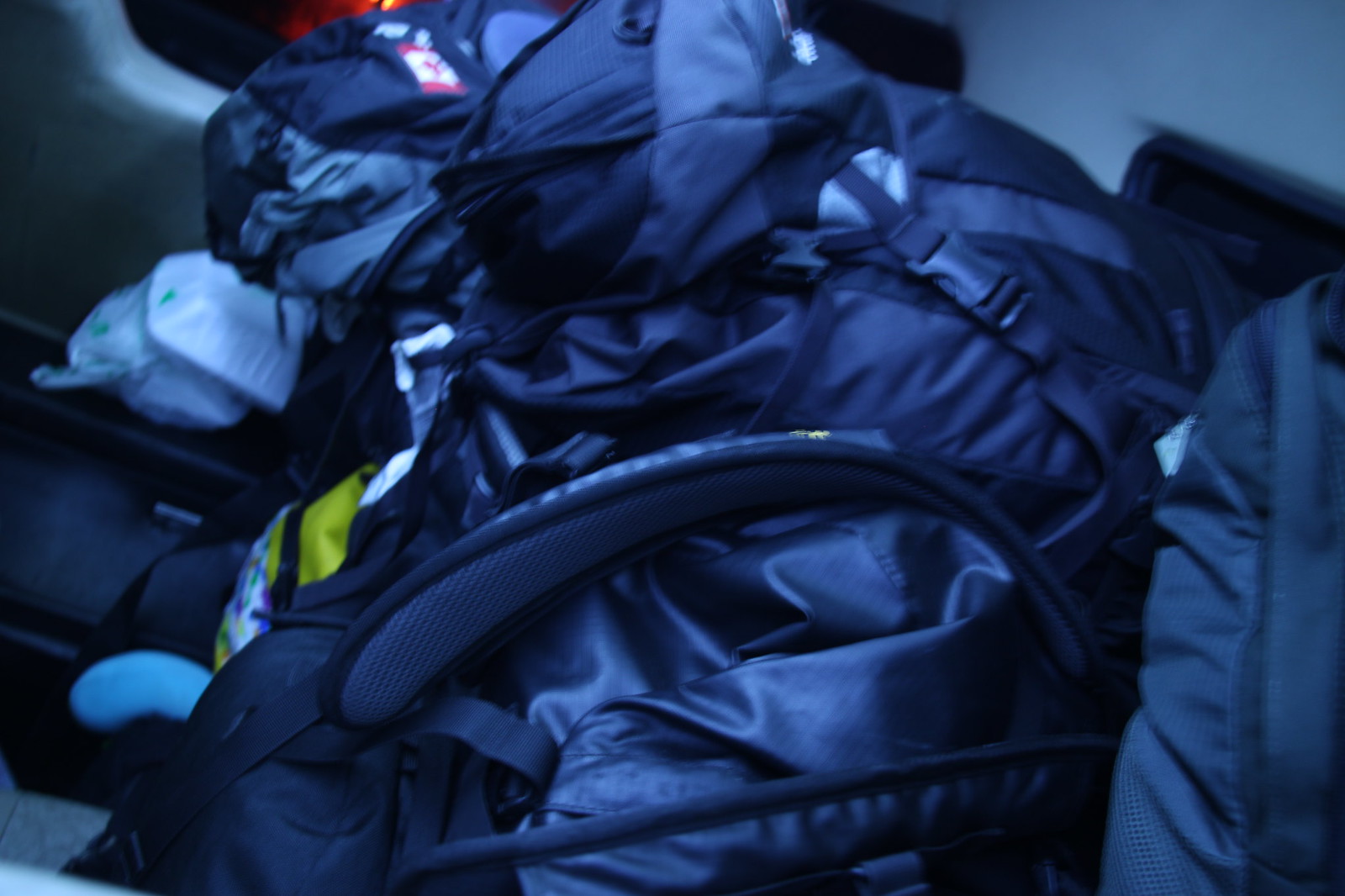The image is a poorly lit and blurry colour photograph with a dark tone, making it challenging to identify all elements with precision. It appears to be a very close-up shot, adding to the ambiguity. The top right of the image shows a backpack complete with a front strap featuring a clasp and elasticated pockets designed for items like water bottles. At the centre of the image, there is another strap, possibly from a different backpack, curving in an arc. On the right-hand side, we see part of what might be another bag or an article of clothing, although it is partially cut off and unclear. Scattered across the left-hand portion of the image are several items that seem to be spilling out from the backpacks. Due to the blurriness, these items are indistinct; they could be wrapped in plastic or resembling polystyrene food containers but are not clearly visible.

Further complicating identification, the background hints at a window with a white frame, potentially situating the scene inside a vehicle, possibly a car or an airplane. This window outline is dark and contributes to the overall unclear context.The left of the frame holds what might be two Styrofoam food containers, reinforcing the idea of food items among the clutter. Additionally, a mix of luggage, jackets, and possibly a sleeping bag or blanket adds to the visual confusion, all appearing as a jumble of darker mesh materials. A small, yellow object is also noticeable in the mix. The overall scene seems to depict a tightly packed, cluttered space—perhaps an interior of a vehicle with someone resting among their belongings.